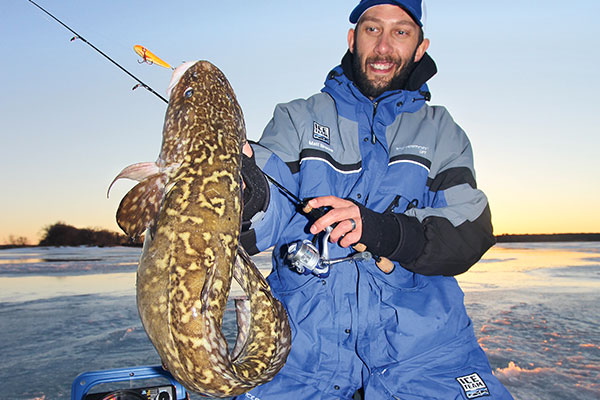In this nature photograph, an ice fisherman, identified as a white man with a beard and a smile, is dressed in a blue cold weather suit with a sweatshirt underneath and a ball cap that reads "Ice Team." He proudly kneels on an ice lake at sunset, holding up a large, tan fish adorned with lighter, mottled gold designs and a yellow hook and bait in its mouth. The fish's curled tail and impressive size add to the scene's dynamic composition. Beside the fisherman, a fishing rod rests in his left hand, and a fishing box can be seen nearby. The backdrop features a serene ice lake with slight rippling water, an island, and a sky that transitions from deep blue to a warm yellow-orange hue as the sun sets, giving an idyllic glow to the entire setting.